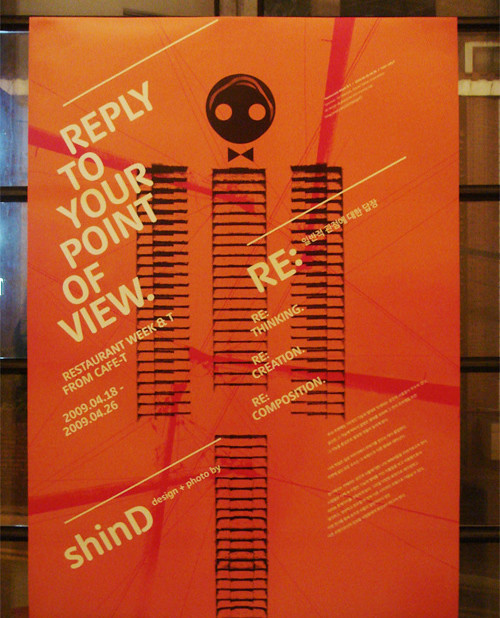In this image, we see a contemporary poster prominently displayed in the center, with a backdrop of wooden material suggesting it may be leaning against some shelving or mounted on a wall. The poster itself features an abstract representation that resembles a robot, consisting of a brown circular head with two eye-like circles and a bow-tie shape formed by two triangles. The body and limbs appear to be stacks or lines, artistically rendered in shades of orange with red streaks.

The text on the poster is angled at about a 45-degree angle to the right. The large, white letters on the left read, "Reply to your point of view, Restaurant Weekend Tea, from Cafe T, 2009-04-18 to 2009-04-26." Additional smaller text includes "Shin D Design" and "Photo by," followed by partially legible text beginning with "R-E:" potentially indicating words like rethinking, recreation, or recomposition. There is also a tiny, illegible paragraph in very small print at the far right of the poster. The overall setting of the image appears to be indoors, with the poster's vibrant and abstract design drawing immediate attention.